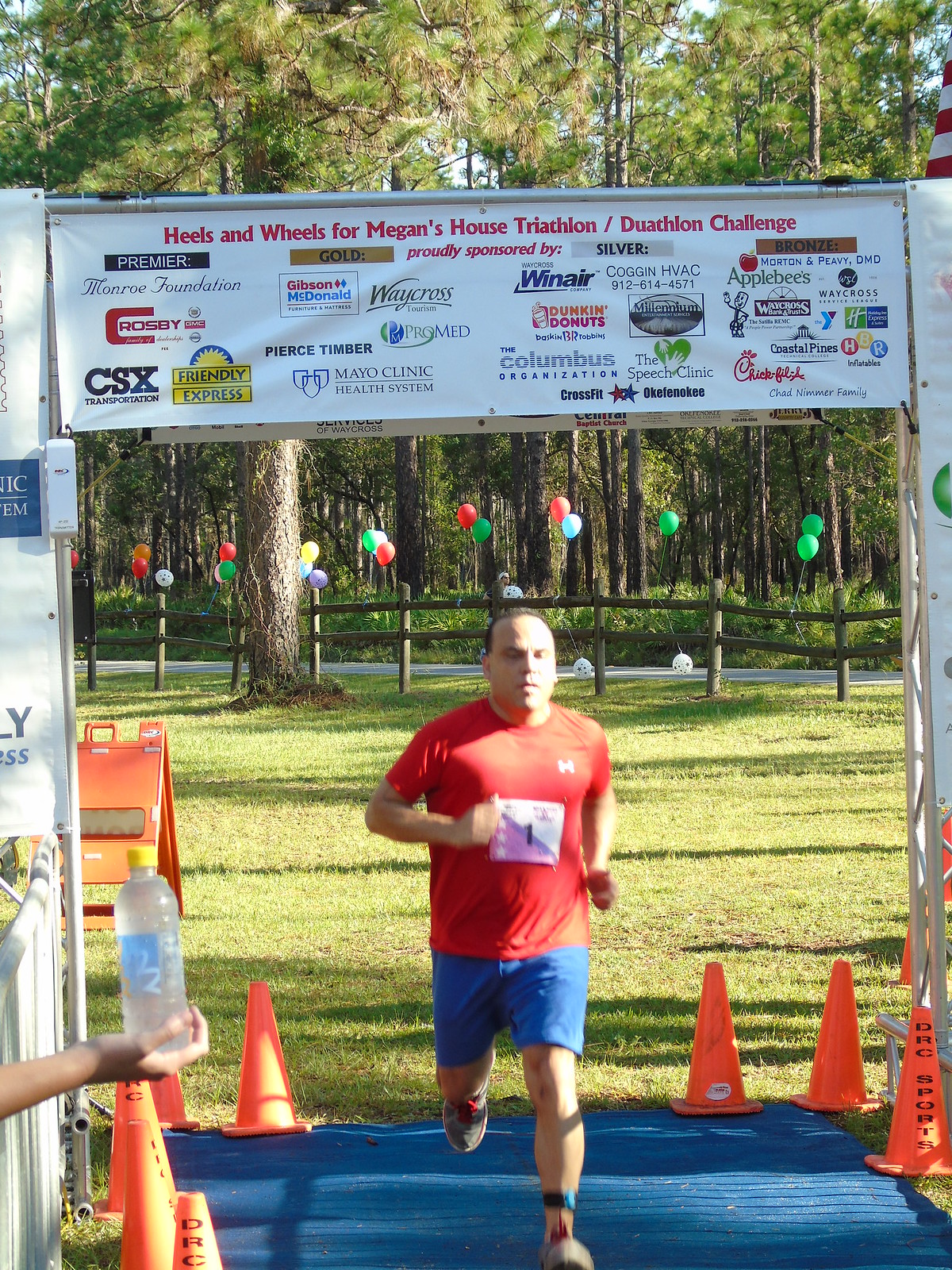The image captures the dynamic moment of a jogger crossing the finish line at a race event set in a scenic park. The backdrop reveals lush green grass, a cement pathway bordered by a rail split fence, and tall spruce trees. Balloons are tied along the fence, adding a festive atmosphere. A man with very short hair, wearing a red Under Armour t-shirt with the logo on the left chest and blue shorts, is seen running towards the banner marking the finish line. His shirt displays the number "1" pinned to the front. He is stepping on a blue mat, indicating the precise moment of his finish. To his left, a Caucasian hand extends a cold bottle of water, suggesting post-race refreshment. Orange caution cones are scattered around the scene. The finish line arch, adorned with the words "Heels and Wheels for Megan's House Triathlon/Duathlon Challenge," lists numerous sponsors, including CSX Transportation, the Mayo Clinic Health System, Gibson McDonald, and many more. The sunlight casts long shadows, indicating it's late afternoon.